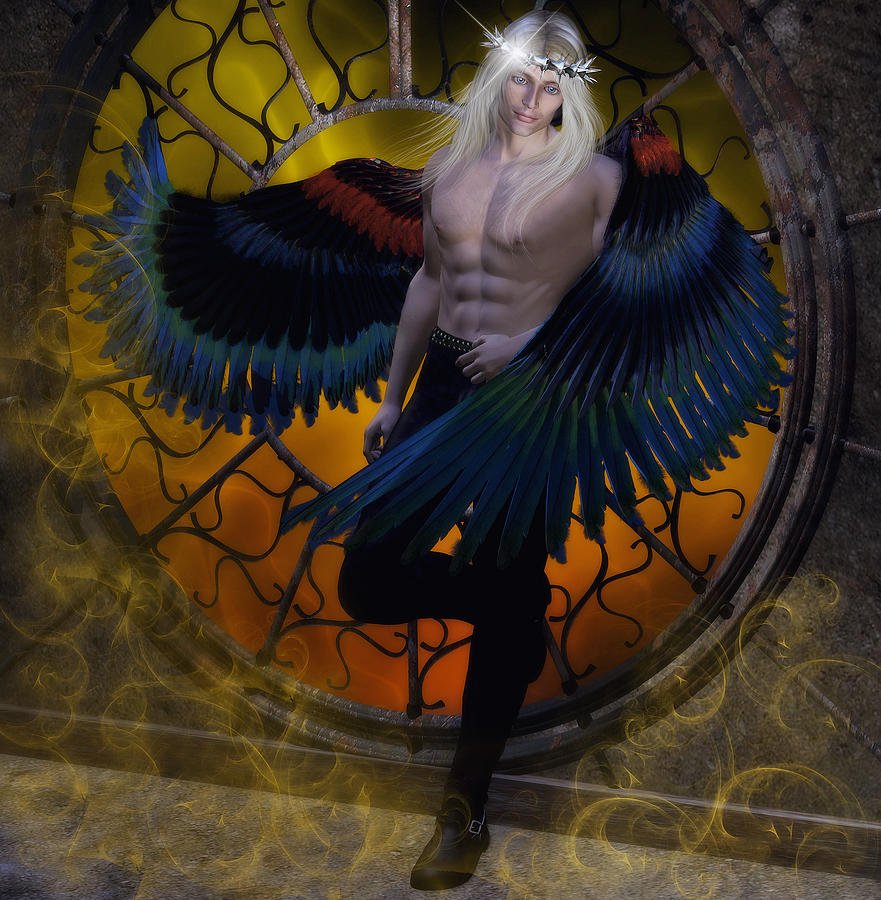This detailed illustration features a shirtless, muscular man with long blond hair, adorned with a shining crown of thorns. He stands in front of a circular window that is segmented by an ornate iron grate into equal sections. The window offers a view of a dark, ominous sky tinged with green and orange hues. The man, who appears to be leaning against the window, has large parrot wings sprouting from his back, vividly colored in shades of blue with hints of red and black. His right leg is bent at the knee, resting against the wall behind him. He holds the buckle of his black pants, which are tucked into boots. The figure's light-colored eyes gaze downward to the left, giving him a silly look as he poses. The room is filled with transparent, swirling gold wisps, adding a mystical ambiance to the scene.